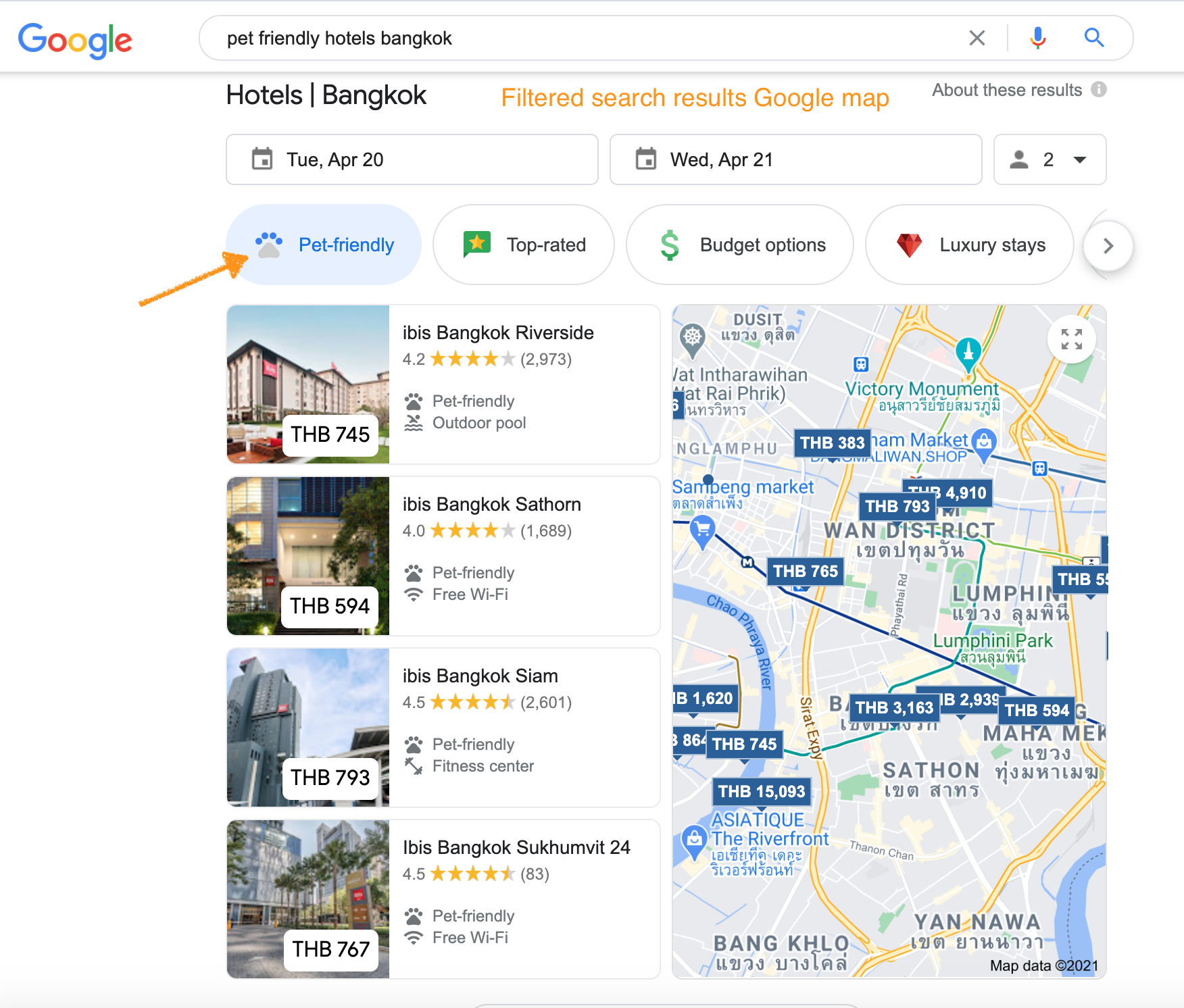The screenshot depicts Google search results for "Pet Friendly Hotels Bangkok." At the very top of the page, a thin light gray horizontal line runs across the width, below which lies a white header. On the left side of this header is the iconic, multicolored Google logo. Moving rightward through negative space, the header features a rounded URL bar with a thin light gray outline, housing the search query "Pet Friendly Hotels Bangkok" in left-justified black text. 

Adjacent to the URL bar on the right is a small cluster of icons: a dark gray "X" for clearing the search, followed by a light gray vertical separator, a multicolored microphone icon for voice search, and finally, a blue magnifying glass icon to initiate the search.

Below this header, a thin light gray shadow is cast onto the main body of the page, which has a white background. In the upper left corner of this section, the word "Hotels" is displayed in black text, followed by a vertical separator. To the right of this, in bold orange text, are the words "Filtered Search Results Google Map." Further to the right, there is a medium gray label stating "About These Results," accompanied by a light gray circle with a white lowercase "i" inside, indicating an information icon.

Underneath this informational section, three text entry options form a single row. The first two entry options are wider and feature dark gray calendar icons on their left sides. The first one reads "Tuesday, April 20th," and the second reads "Wednesday, April 21st." The third, smaller entry option, has a dark gray profile icon to its left, followed by the black numeral "2," and a black downward-facing triangle.

Directly beneath these entries, several filter options are prominently displayed: "Pet friendly," "Top rated," "Budget options," and "Luxury stays." An orange arrow points specifically to the "Pet friendly" option, drawing attention to this particular filter.